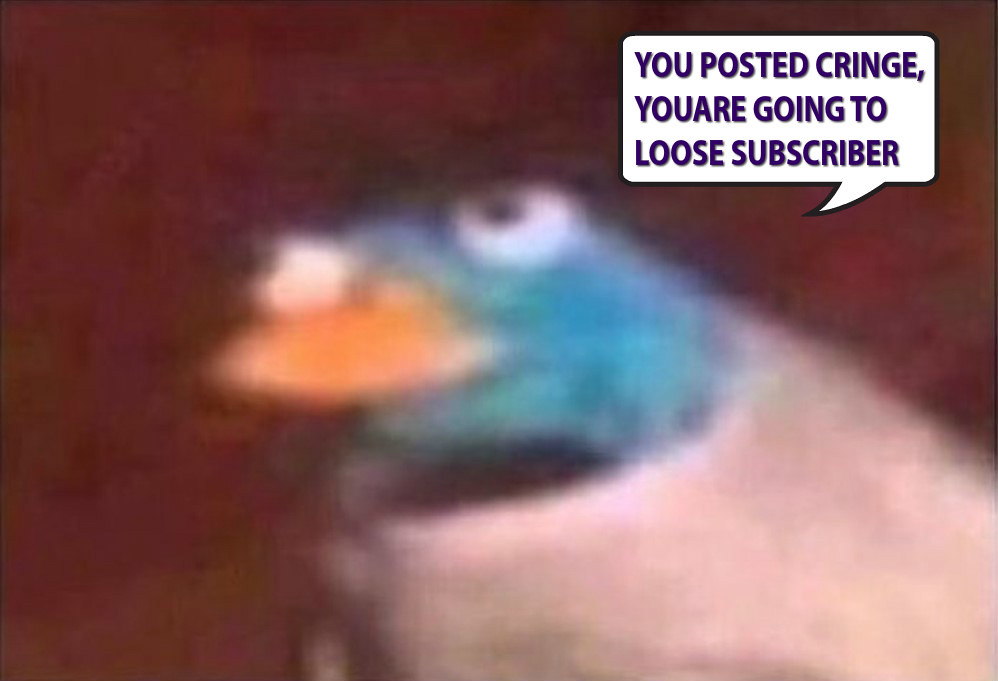This image is a very blurry graphic with a reddish-brown, maroon background featuring a creature that closely resembles a bird. The bird has large, spherical white eyes with black pupils and a long, orange beak. The area around its face is blue, and there is black on the top of its head, which could be feathers or possibly something it is wearing. Its body appears quite large and is mostly white, giving the impression it might be wrapped in something like a white sweater. The bird looks somewhat sad and depressed. There is a speech bubble emanating from the right side of the bird's head, containing the text "YOU POSTED CRINGE. YOUARE GOING TO LOOSE SUBSCRIBER." The message includes several errors: "YOUARE" should be two separate words, "LOOSE" should be "LOSE," and "SUBSCRIBER" should be plural.